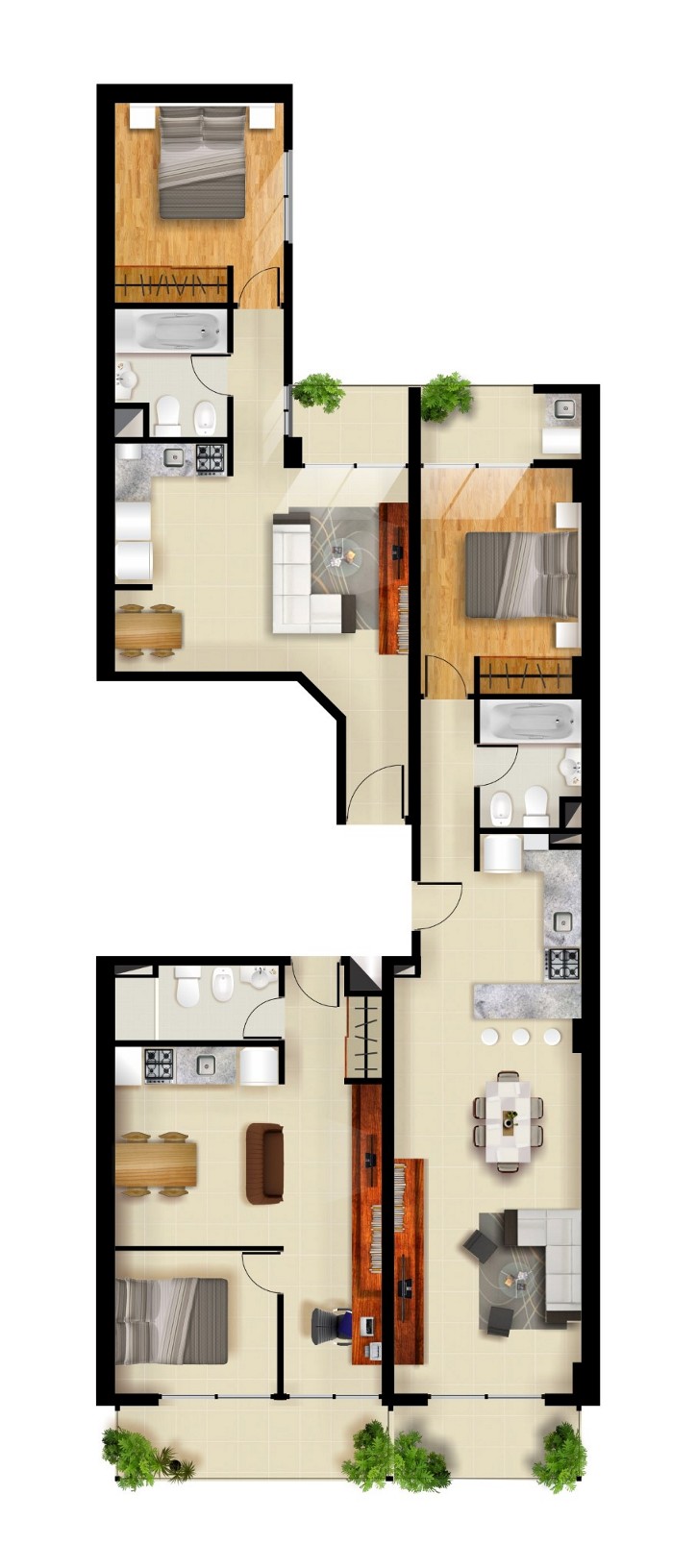This is a detailed top-down design layout of a spacious residence, which appears to be a cluster of three connected apartments. Each apartment features distinct living spaces and conveniences.

**Apartment 1:**
- **Bedrooms:** 1
- **Bathrooms:** 1, directly accessible from the bedroom
- **Other Features:** A large kitchen with space for a dining table and direct access to a small patio.

**Apartment 2:**
- **Bedrooms:** 1
- **Bathrooms:** 1, directly accessible from the bedroom
- **Other Features:** A large dining area, a spacious living room with access to a common large patio.

**Apartment 3:**
- **Bedrooms:** 1
- **Bathrooms:** 1
- **Other Features:** A living room/dining room combination and a small kitchenette, with a private patio accessible from the bedroom.

Central to the design is a large common patio accessible from both the second apartment’s living room and bedroom, enhancing communal living. Each apartment has its own dining area, ensuring enough space for individual household needs, while cleverly integrating the three into a cohesive, larger home.